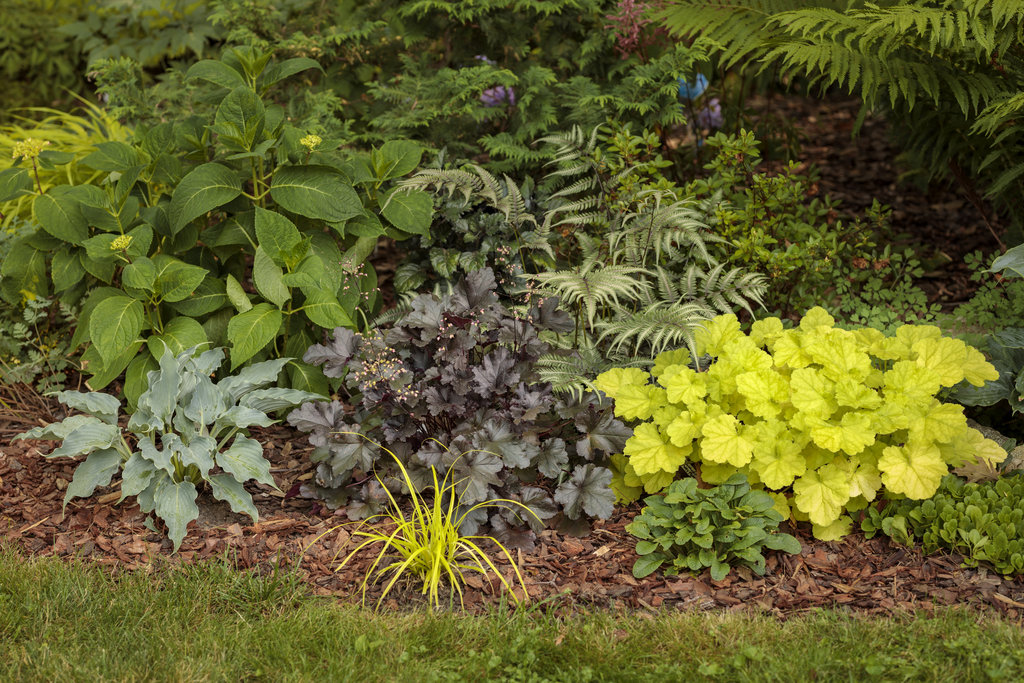This is a photograph of a vibrant garden bed. At the bottom of the image, there's a foreground of neatly trimmed green lawn, giving way to a neat border of bright mahogany brown mulch. This mulch bed hosts an array of distinct and colorful plants. To the left, there is a lush, bright green plant with circular leaves, followed by a striking lime yellow-green bush. Adjacent to it is a dark, purpley-green bush with somewhat velvety texture, creating a beautiful contrast. In the center stands a very light green clump of grass with slender blades. Further to the right, a bold, light green bush with broad, robust leaves can be seen, possibly adorned with some yellow flowers. Behind these, in the background, the garden bed transitions into a symphony of blue and purple flowers interspersed with varied foliage, including fern fronds and spiky leaves, contributing to the garden's lush appearance. This detailed arrangement highlights the diverse textures and colors, making the garden a captivating sight.